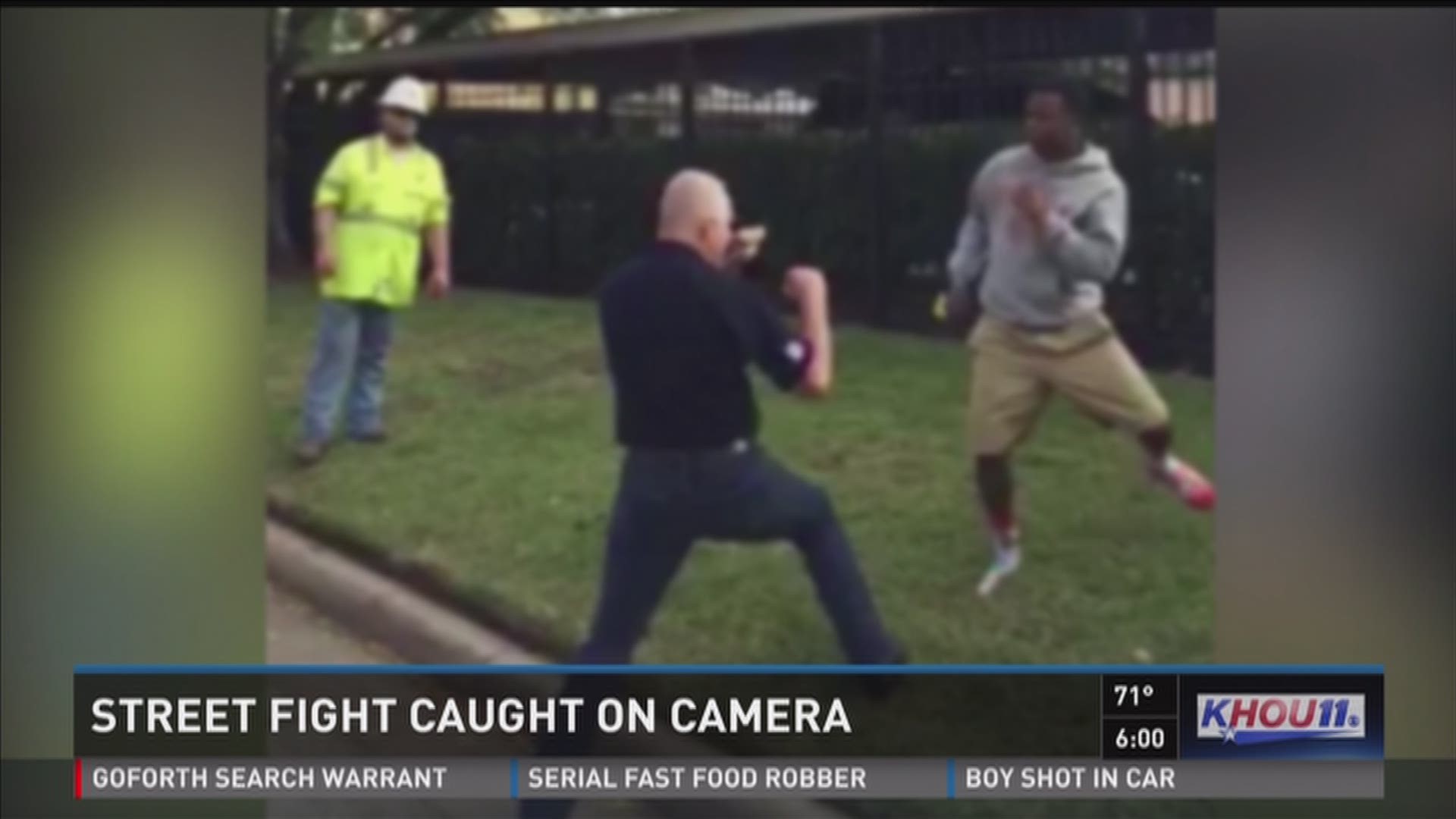In the image, two men are poised for a fight in a grassy area that seems to be a yard or near a roadside curb. One of the men, a bald white Caucasian dressed in a blue pullover shirt and denim jeans, has his fists raised defensively. Opposite him stands a black man in a gray hoodie, tan shorts, and red tennis shoes, also ready to fight with his fists up. Observing the scene is a man who appears to be a construction worker, identifiable by his bright lime green vest with safety tape and a white helmet. The background features a building with ivy creeping up its facade, and the sides of the image are blurred in gray tones. At the bottom of the image, the text "Street Fight Caught on Camera" is displayed, followed by "K hour 11," suggesting that the altercation was broadcasted on television.